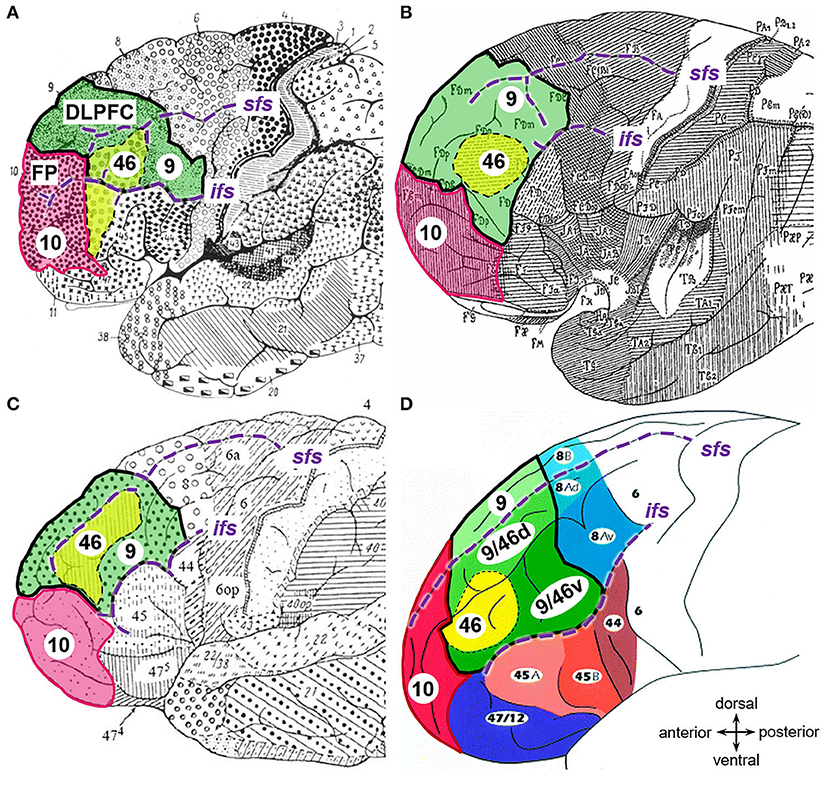This composite image consists of four distinct diagrams, each illustrating different aspects of the brain. These diagrams are arranged in a 2x2 grid and are labeled A, B, C, and D sequentially from top left to bottom right.

Diagram A presents a detailed illustration of the brain with various sections marked by different textured dots and colors such as green, red, and yellow. Specific regions are numbered and labeled, including sections 9 (DLPFC), 10 (FP10), and 46. Each of these regions is distinctly shaded—section 9 in green, 10 in purple, and 46 in yellow.

Diagram B highlights the combined sections of areas 9 and 46 shaded together in green and yellow, and section 10 in purple. The diagram features grayed-out areas, with certain sections like regions 9, 10, and 46 brought to the forefront through their color coding.

Diagram C, similar to A, showcases the brain with varied textures and colored sections in green, yellow, and red, each labeled with numbers for clear identification.

Diagram D offers a more simplified view with clear black outlines of the brain and colorful regions within it. It serves as a map, indicating orientations with 'dorsal' at the top, 'ventral' at the bottom, 'anterior' to the left, and 'posterior' to the right. Numbers such as 46, 10, and others are clearly annotated on the diagram.

All four diagrams collectively provide a comprehensive view of different brain regions, their textures, and their functions, making the anatomical and functional organization clear through color-coding and labeling.